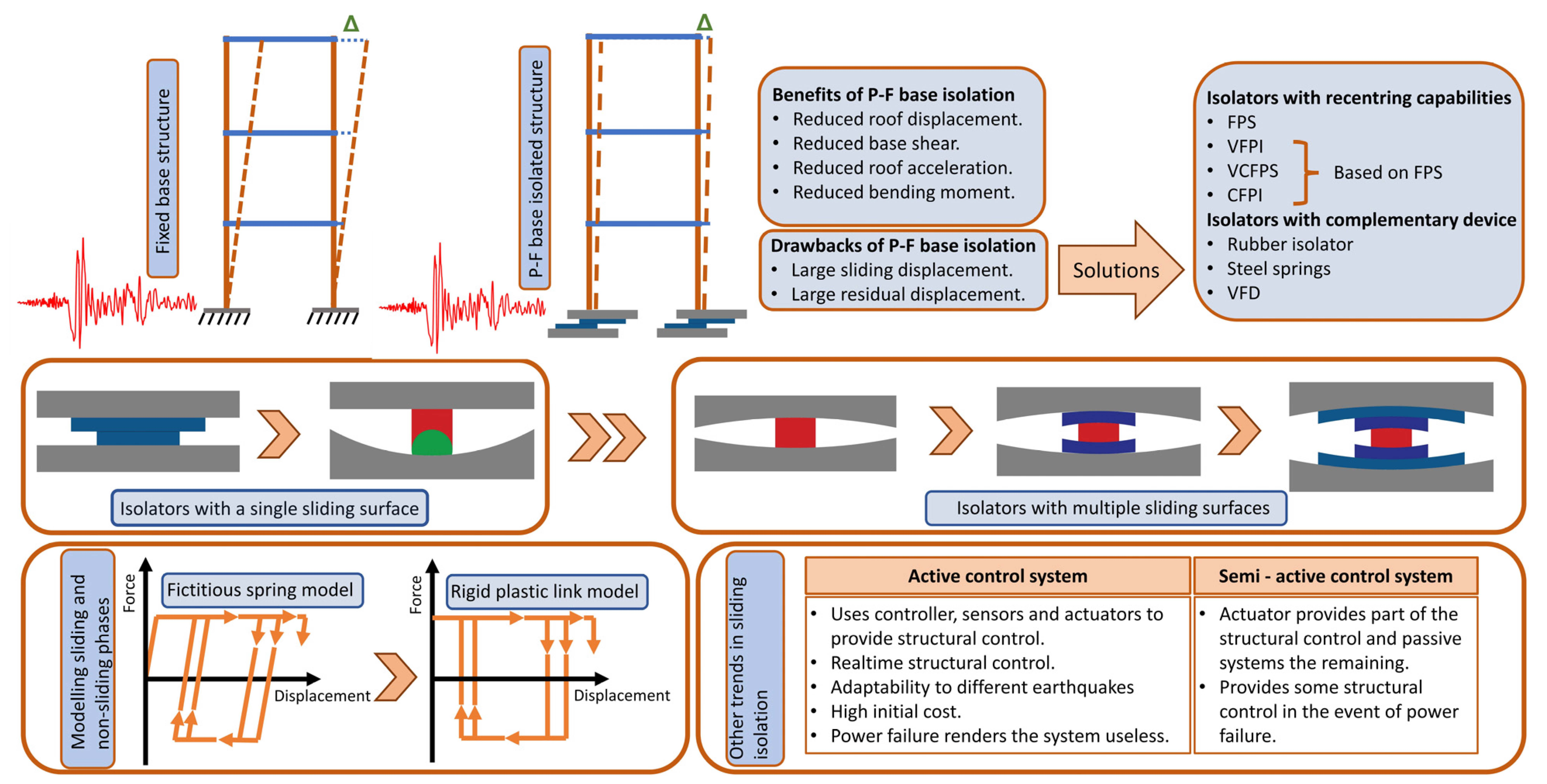The diagram is a highly detailed infographic depicting a machinery process, likely used as an educational tool for a science class project. The top part of the diagram features two structural frames labeled "Fixed Base Structure" and "PF Isolated Structure," distinguished by orange and blue lines, with some blue dotted lines. Boxes of text provide insights into the "Benefits of PF Base Isolation" and "Drawbacks of PF Base Isolation," accompanied by proposed solutions. A pathway runs horizontally across the center, illustrating "Isolators with a Single Sliding Surface" that transition into "Isolators with Multiple Sliding Surfaces," marked by arrows. The bottom section includes various models, such as a "Sliding Model," "Non-Sliding Phases," "Fictitious Spring Model," and "Rigid Plastic Link Model." Additionally, a box in the lower right corner details the features of "Active Control Systems" and "Semi-Active Control Systems," enhancing the comprehensive overview of this complex system.